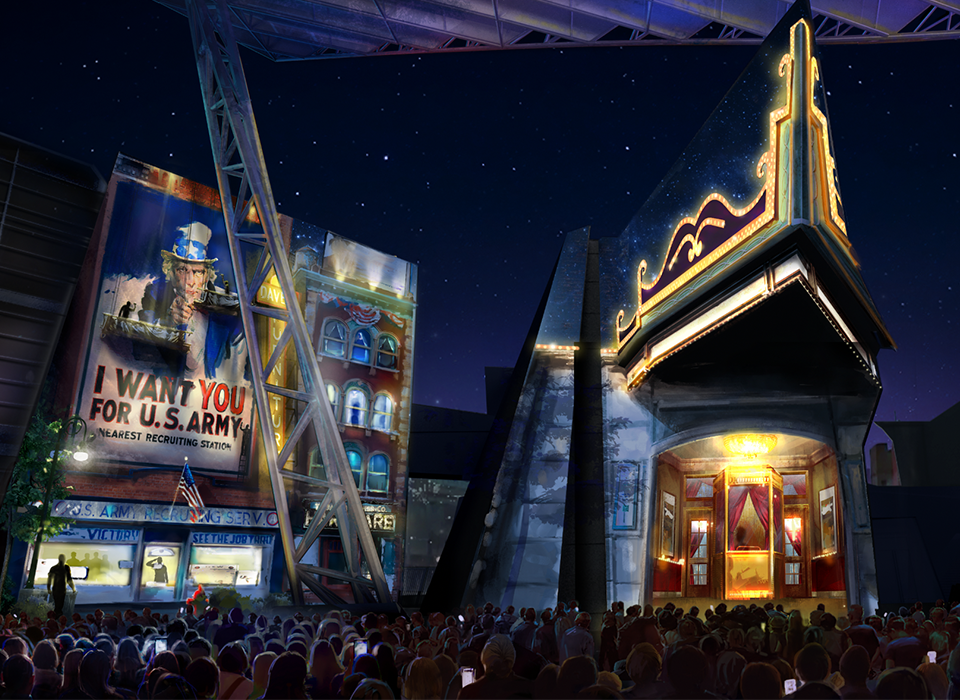The image depicts a generated or stylized nighttime scene with a large crowd of people standing beneath a starry sky. The crowd appears to be visiting what seems like a movie set or temporary outdoor structure. They are gathered in front of two distinctly old-fashioned buildings. One building resembles an antique movie theater, brightly lit with a vintage box office where a person might be ready to sell tickets. The adjacent building is a U.S. Army recruitment center, prominently featuring a classic Uncle Sam poster with the slogan "I Want You for the U.S. Army" and some scaffolding partially obstructing it. Many in the crowd are holding smartphones, capturing the scene, with their faces and devices faintly illuminated by the ambient light reflecting off the structures and streetlights. The setting exudes an atmospheric, old-world charm, blending historic elements with a modern crowd.